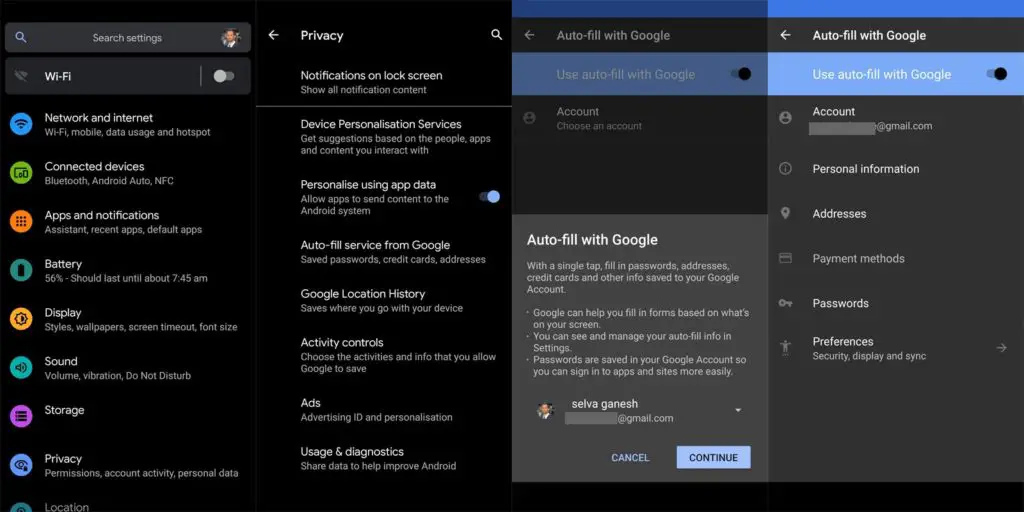This image is a detailed screenshot of a phone's settings interface, specifically focusing on the Wi-Fi section of a website. The screenshot captures the settings page where various tabs like “Search Settings,” “Wi-Fi,” and others are visible. The user has navigated to the “Privacy” tab within the Wi-Fi settings. The “Privacy” section displays multiple subsections, each represented by individual tabs.

The highlighted tab is associated with “Autofill with Google.” Within this section, there is a description explaining the autofill feature accompanied by the option to enable or disable it. Additionally, it showcases a partially-obscured email address, likely for privacy reasons. Prominently displayed are the options “Cancel” and “Continue,” suggesting the user can either cancel the action or proceed with enabling Google Autofill.